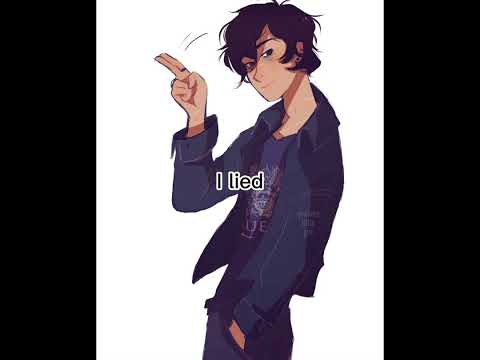In this image, a cartoon character is depicted with a highly detailed and expressive pose. The character, dressed in a matching purple ensemble consisting of a jacket, t-shirt, and trousers, exudes a cool and nonchalant demeanor. The character is positioned facing towards the left side of the frame, with their left hand casually tucked into their pocket. Although the character's body is oriented to the left, their head is slightly tilted forward, creating an engaging, dynamic posture.

The character's right hand is raised, with two fingers—the index and middle fingers—extended in a pose reminiscent of a peace sign, pointing towards the top left corner of the image. The remaining fingers, including the pinky, ring finger, and thumb, are bent inward, resting against the palm. This gesture adds a layer of playful confidence to the character.

A notable feature of the character is their vibrant purple hair, which mirrors the color of their attire. The hair is curly and cascades gently around the face, slightly covering the cheeks, complementing the character’s overall aesthetic.

Superimposed on the center of the image is a bold text that reads, “I lied.” The text is black with a white outline, making it stand out prominently against the white background. The image is framed by physical black bezels on the left and right sides, which are slightly thick and further emphasize the central subject.

The overall composition, with the monochromatic purple outfit, expressive hand gesture, and striking text, creates a memorable and vivid visual narrative.